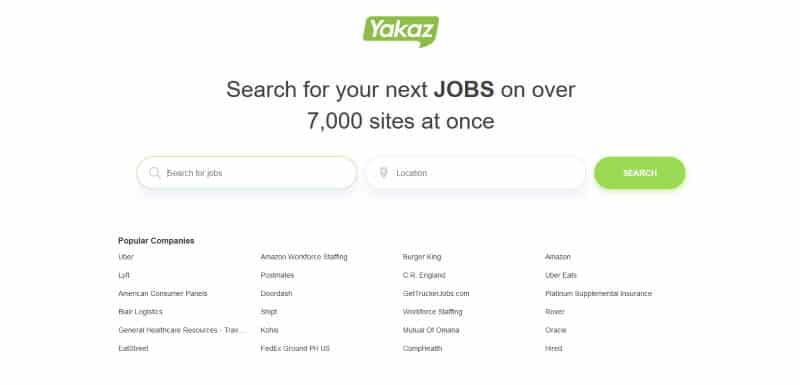The image depicts a web page for "YAKAS" featuring a distinctive lime green logo at the top. Below the header, there's a prominent tagline in black text that reads, "Search for your next job on over 7,000 sites at once." The page highlights a central search functionality with a search box labeled "Search for jobs," accompanied by a white magnifying glass icon. Additionally, there is a location filter allowing users to input their city or town, plus a green search button to initiate the job search.

Directly below these search tools, the page lists "Popular Companies," showcasing a selection of notable employers such as Uber, Lyft, Burger King, Amazon, FedEx, Uber Eats, and Oracle among approximately 25-30 other companies. The overall page layout features a clean, white background with black text and white search boxes. The primary objective of the site is to facilitate comprehensive job searches across a vast array of potential employers, ensuring users can efficiently find employment opportunities.